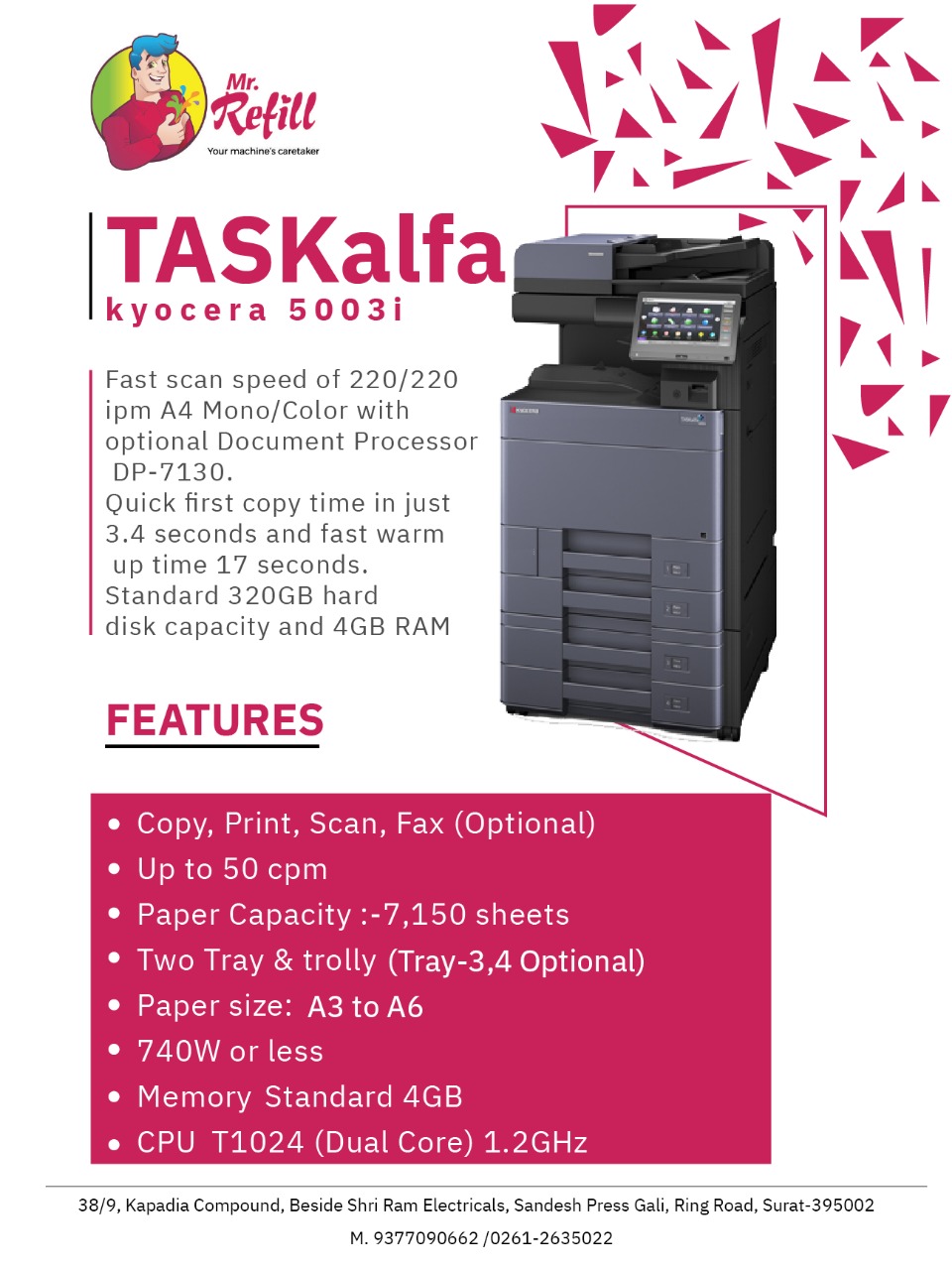The advertisement, displayed in portrait mode, showcases a high-end, industrial-sized office printer and scanner. The image is divided into two sections: an upper white half and a lower pink half. In the upper left corner, a colorful logo of a man, labeled "Mr. Refill," is accompanied by geometric patterns. The main visual on the right side in this section is a large office printer with several trays, emphasizing its commercial utility. 

To the left of the printer image, in pink text, is the model name "Taskalfa Kyocera 5003i," followed by black text detailing its impressive specifications: a rapid scan speed of 220 IPM for A4 mono and color documents with an optional document processor DP-7130, a quick first copy time of just 3.4 seconds, and a fast warm-up time of 17 seconds. The printer boasts a standard 320GB hard disk capacity and 4GB of RAM.

In the pink lower half, white text over a red box lists multiple features, highlighting the printer's advanced copying, printing capabilities, memory, and CPU performance, all of which underline its efficiency and suitability for a high-demand office environment.